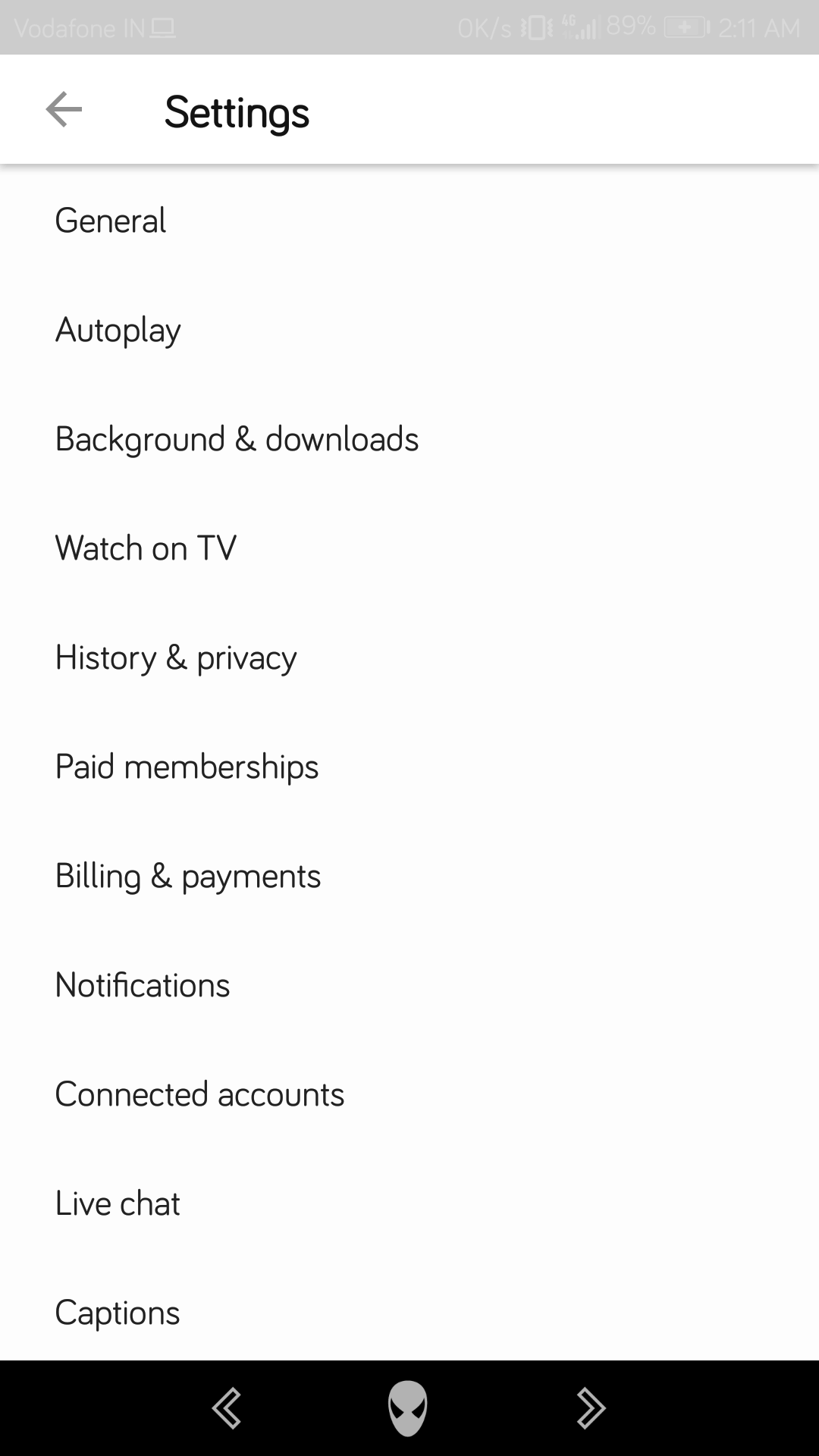A cell phone screen displays the "Settings" menu, with the word "Settings" prominently written in black at the top against a white background. At the very bottom of the screen, there is a distinct black rectangle featuring white forward and back buttons on either side of a small Spider-Man face icon in the center. 

Beneath a faint gray line near the top of the display, a vertical list of options is shown, beginning with "General," followed by "Autoplay," "Background and Downloads," "Watch on TV," "History and Privacy," "Paid Memberships," "Billing and Payments," "Notifications," "Connected Accounts," "Live Chat," and finally, "Captions."

At the very top of the screen, a gray rectangle spans from the left to the right edge, housing several icons and informational text. It indicates network provider "Vodafone IN," a TV icon, and additional details on the right side, which read "OK/S" and the time "2:11 a.m."